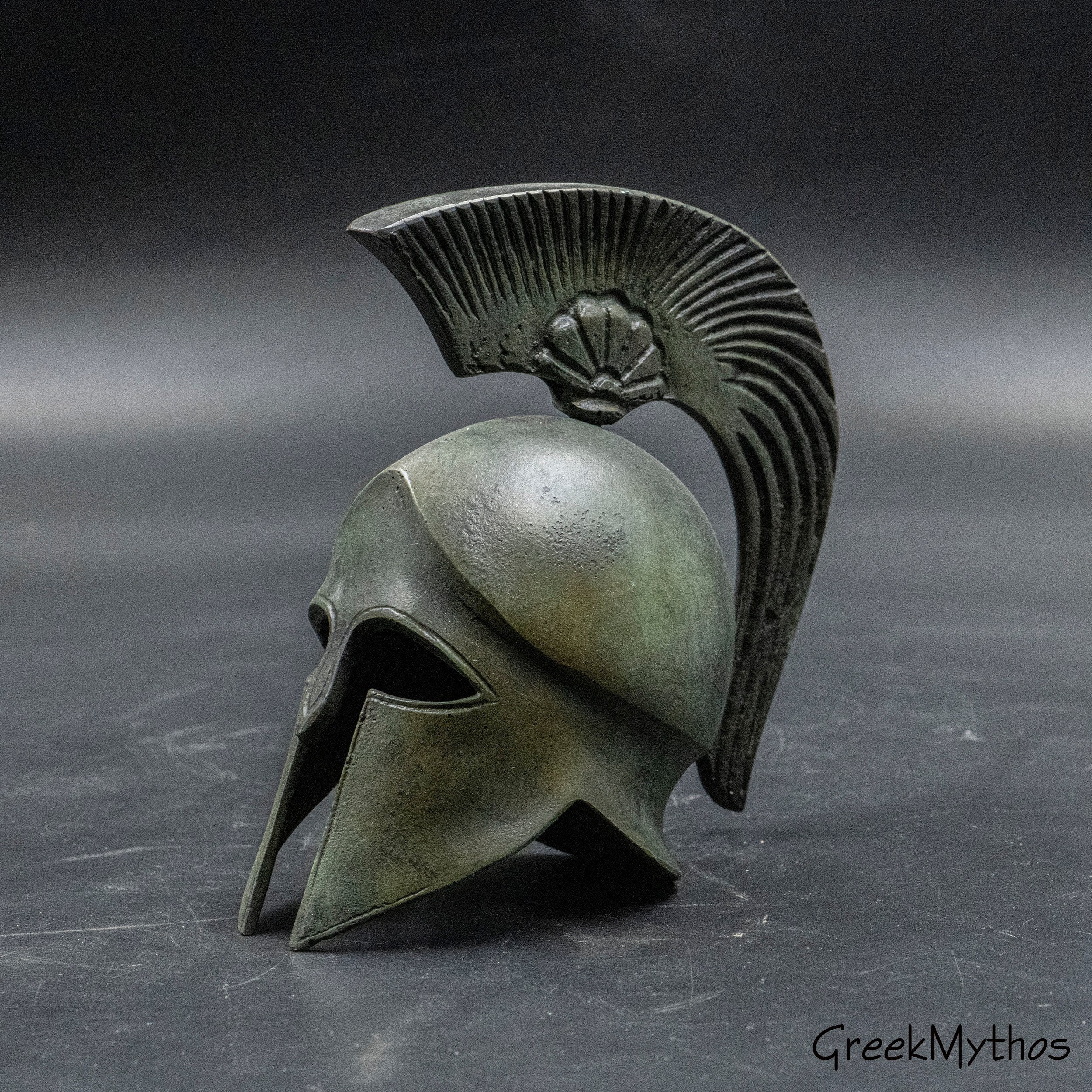This is a detailed photograph of a bronze Greek gladiator-style helmet displayed on a plain, dark gray surface, possibly slate or concrete, against a matching gray background. In the lower right corner of the image, the text "Greek Mythos" is printed in black sans serif font. The helmet features prominently in the center with oval eye holes that are pointed at the outer edges, providing limited visibility. Below the eye cutouts, a vertical nose guard descends to the middle of the face, offering partial coverage for the nose. The helmet's sides curve down to form pointed pieces over the cheeks. At the top, a decorative bronze piece resembling a feather or mohawk curls from the front of the forehead to the back of the helmet, adding an ornamental touch to the functional design. The metal appears aged, with hints of green patina suggesting its historical character.